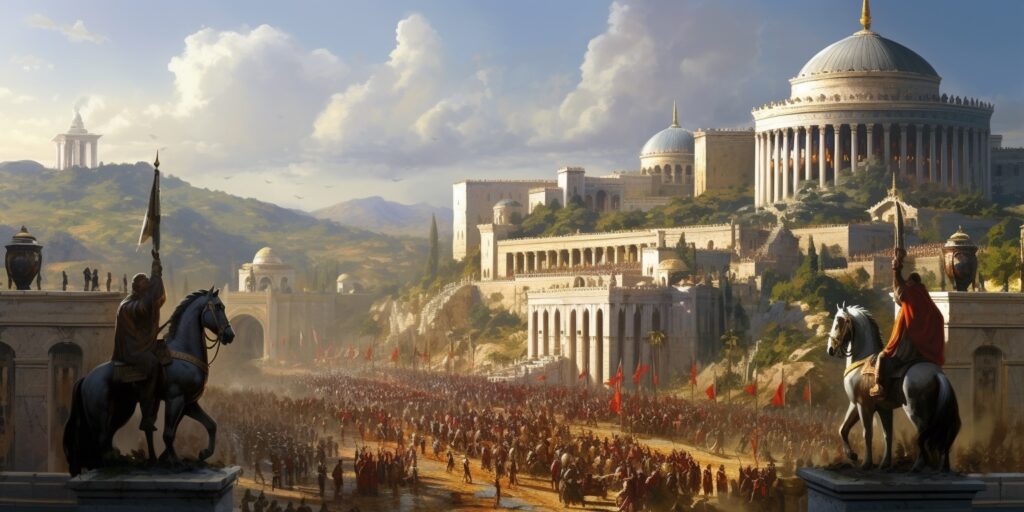The image depicts a meticulously detailed scene of an ancient civilization, potentially Greek or Roman, characterized by grand architectural structures and a bustling crowd. Dominating the right side is a collection of impressive buildings featuring blue-domed, rounded roofs and golden pillars, situated on a verdant hillside adorned with trees. Central to the image, a large procession or army holds up numerous red flags as they march towards the foreground. 

In the forefront, two statues or men on horseback are positioned on pedestals. The left figure rides a dark gray horse, while the right figure is mounted on a white horse with a black tail, both bearing flags or staffs. To the left of the procession is another building with people engaged in activity, such as handling a pot. 

The background showcases another hill with a significant structure atop it, likely a monument or altar, set against a blue sky with scattered clouds. Light illumination suggests the sun is positioned off-screen to the left. Visually striking, the image blends classical architecture and a dynamic assembly, hinting at a significant event or gathering within this ancient cityscape.